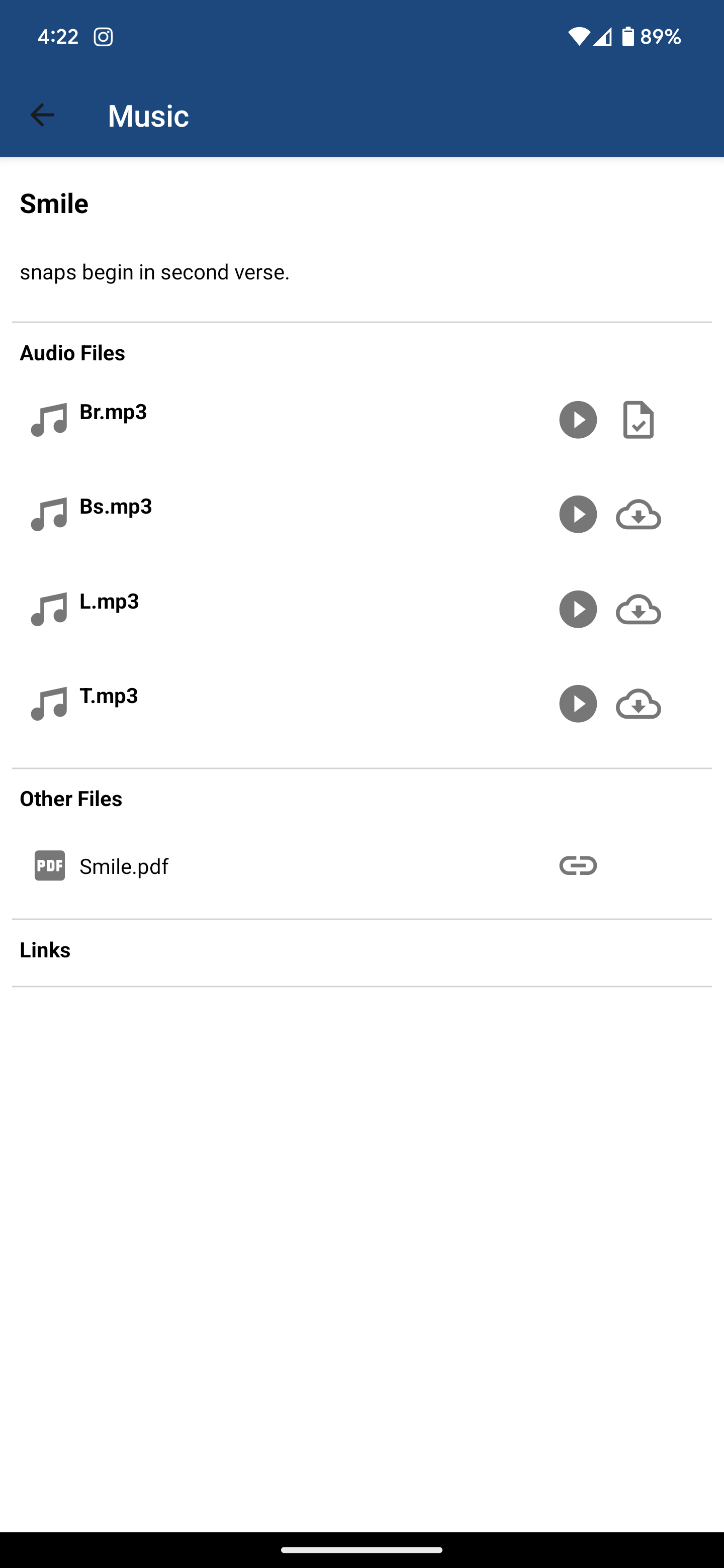This image depicts a smartphone screen displaying an application interface under the "Music" category. At the top of the screen, there is a blue header featuring the current time at 4:22 PM, alongside an Instagram icon to the right. The right side of the header shows white icons indicating the Wi-Fi signal strength (three out of four bars), cellular signal (three out of four bars), and battery level (89%).

On the left side, a black back button is present, and in white text, the word "Music" is displayed. Just below, there is another header that reads "Smile" with a subtext "Snaps begin in second verse." Underneath, "Audio Files" is indicated in black text, followed by the term "Set."

The interface shows four options for audio files, each accompanied by grey musical note icons. The first file, "br.mp3," is marked with a check indicating it has been downloaded. The next three files— "bs.mp3," "l.mp3," and "t.mp3"— feature cloud icons with download buttons, suggesting they have yet to be downloaded. Each file entry has a play button represented by a triangle in a grey circle on the far right.

A thin line separates the audio files section from another labeled "Other Files," which includes a grey box containing "smile.pdf" in white text and a link icon adjacent to it.

Below this, a section labeled "Links" is seen, followed by a considerable amount of white space. At the bottom of the screen, there is a black bar that marks the edge of the phone's display.